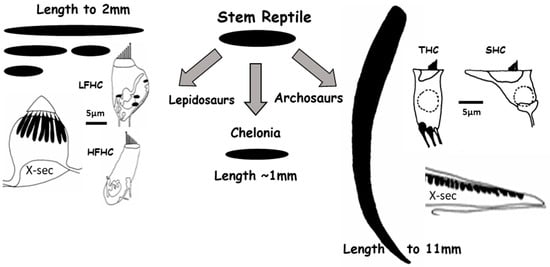The image depicts a detailed black-and-white scientific chart from a textbook, illustrating the concept of a 'stem reptile.' The chart is divided into three sections, each associated with specific measurements and annotations. 

At the top, the central section is labeled "stem reptile," and features a central oval or circular area annotated with “length ≈ 1 millimeter.” Three arrows emanate from this circle, pointing to the words "Lepidosaurs" (left), "Archosaurs" (right), and "Che Ionia" (bottom).

The left section, marked "length ≈ 2 millimeters," includes four small black oval shapes, possibly suggesting various species or anatomical features. Detailed annotations such as "LFHC," "HFHC," and "X-sec" (cross-section) accompany these shapes, indicating specific traits or measurements.

The right section showcases a lengthy black shape, resembling a tooth or elongated object, labeled "length ≈ 11 millimeters." This section further includes three images marked with "THC," "SHC," and "X-sec," each annotated with "5UM," possibly indicating magnifications or scales.

Overall, the chart relies heavily on black and white imagery, combining scientific labels with intricate drawings to explain the anatomical and evolutionary traits of stem reptiles.